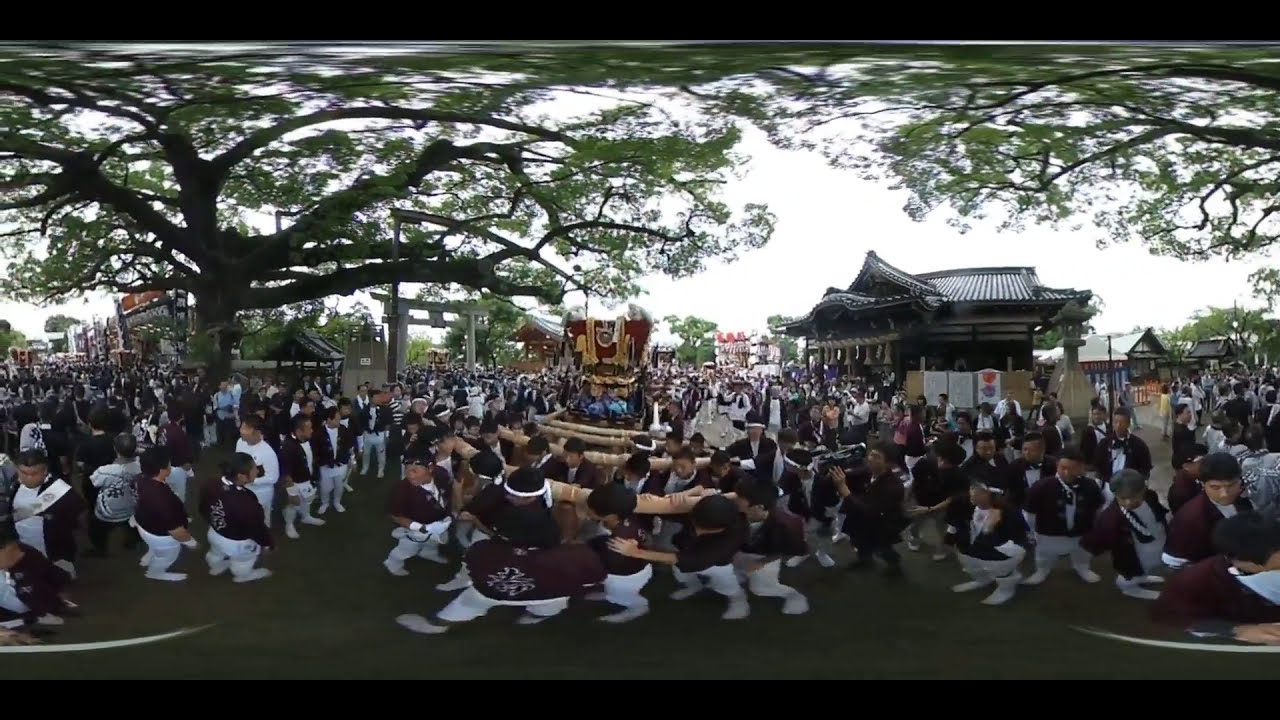The image depicts a very large crowd of people gathered on a solid, light green surface, which resembles grass. Most of the individuals, seemingly all men, are dressed in white pants and black or maroon shirts, with several wearing white headbands. Central to the scene, a group of men are engaged in a competition, carrying four long wooden poles horizontally across their shoulders, spanning over three or four people. They all have black hair and white shoes.

In the background, on the right side, stands an oriental-style building with an arched roof, painted green. The upper right corner shows branches with green leaves extending over the building. On the far left, a large tree with a substantial trunk and heavy, green-leafed branches frames the scene. The sky above the gathering is a solid white, indicating it is possibly daytime. The photograph's setting suggests an outdoor event in an Asian country, enriched by the traditional architecture and the tree-filled environment. The image features no textual elements, and its composition is framed with a solid black border at the top and bottom.